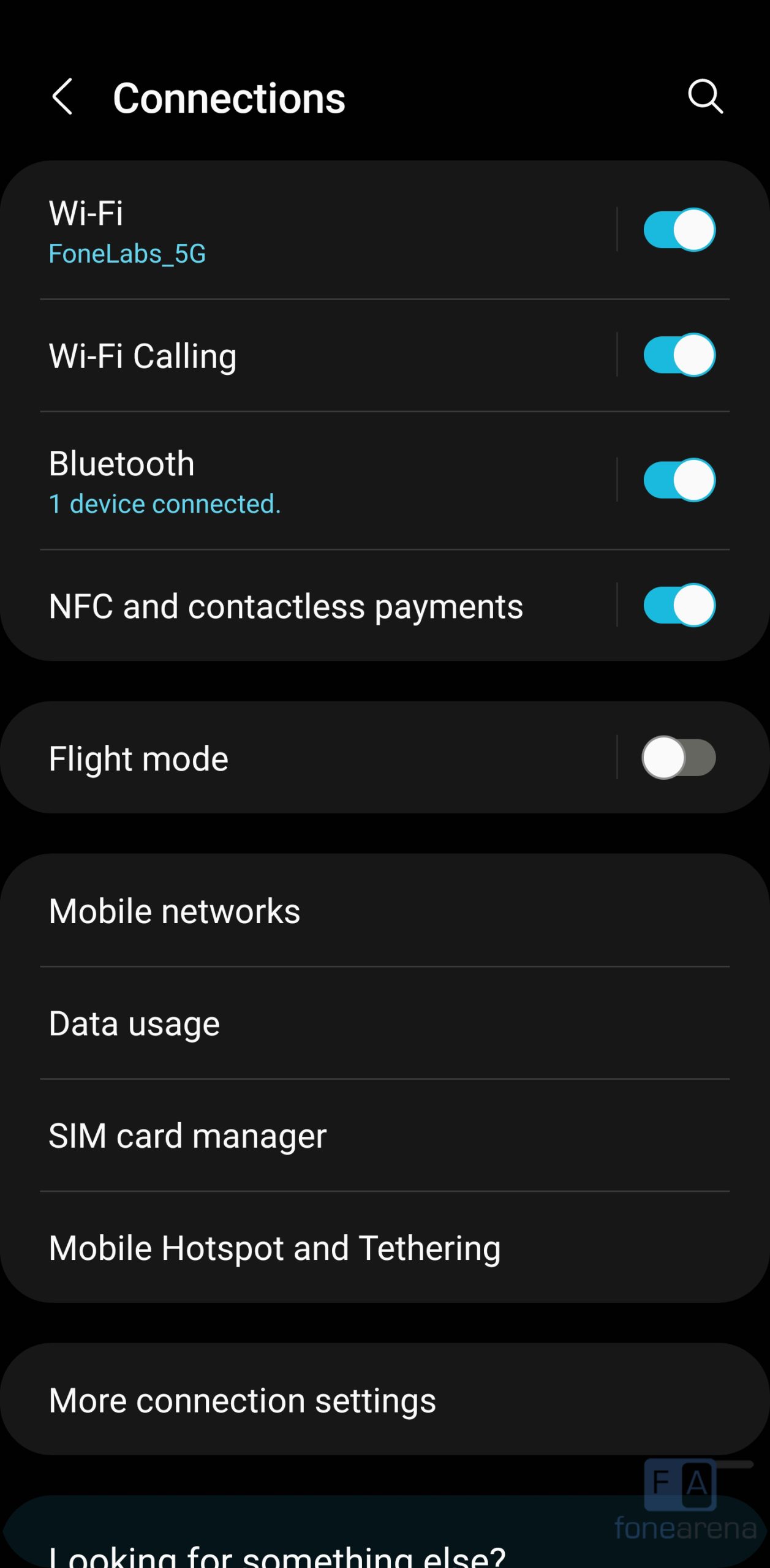"On a black smartphone screen, the top left corner displays a left-pointing arrow followed by the word 'Connections.' On the top right, there is a search icon. Below, 'Wi-Fi' is listed with 'phone labs_5G' highlighted in blue and toggled on. Separated by lines, 'Wi-Fi Calling' is also toggled on in blue. 'Bluetooth' shows 'One device connected,' and is toggled on in blue.

Further down, 'NFC and Contactless Payments' is toggled on, while 'Flight Mode' is not. Additional options listed include 'Mobile Networks,' 'Data Usage,' 'SIM Card Manager,' 'Mobile Hotspot and Tethering,' and 'More Connections.' The lower part of the screen is slightly cut off, obscuring part of the text.

In the bottom right corner, 'Phone Arena' is faintly visible, with an 'F' on a white background and an 'A' on a red background, both partially obscured as if under a gray film. The color scheme throughout includes black, white, blue, gray, and red."